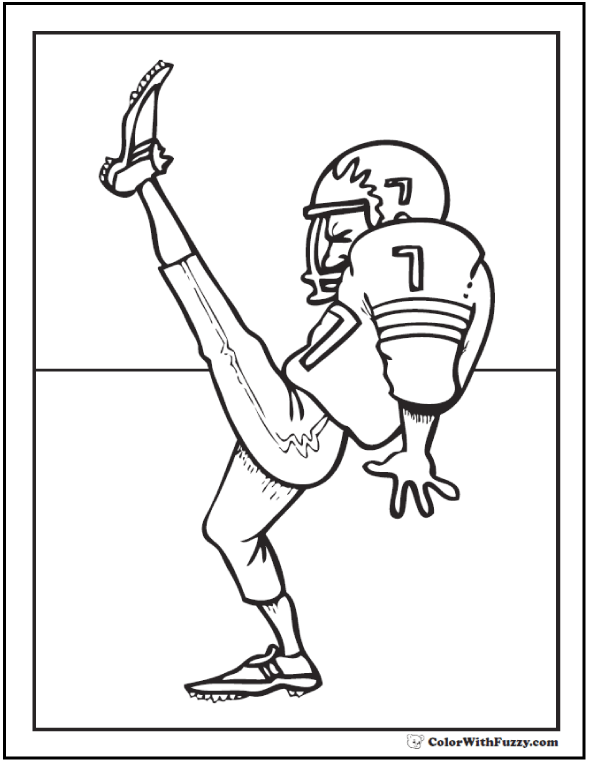This black and white sketch, reminiscent of a coloring book illustration, depicts a humorous caricature of an American football player mid-action. The player, wearing a helmet adorned with the number 7 and football pads, has his left leg dramatically kicked high up into the air, almost reaching the upper left corner of the image—all the while maintaining a rigid posture with his other foot flat on the ground. The cartoonish character has skinny legs and cleats, with a visible stripe down the side of his pants. The scene is minimally detailed, focusing solely on the player, who is surrounded by a black boundary and a horizontal line that divides the image, suggesting the edge of a football field. The sketch is entirely monochromatic, with a stylish yet simple outline that hints at a playful scenario, such as the possibility of the player either just having kicked a football or missing a field goal. The bottom right corner is marked with the text "ColorWithFuzzy.com," indicating that the image is likely designed for coloring purposes.